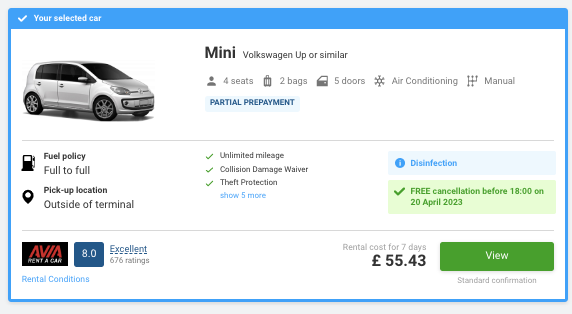The displayed image features a highlighted blue bar indicating the selected car, which is labeled as "MINI, Volkswagen up or similar." Details about the vehicle include seating for four, capacity for two bags, five doors, air conditioning, and a manual transmission. Text in blue mentions "partial prepayment." Adjacent to this is a divider line, followed by information on the fuel policy which states "full to full." The pickup location is specified as "outside of terminal," and it offers "unlimited mileage."

The image includes several green check marks confirming additional features like a "collision damage waiver," "theft protection," free cancellation available before the 18th of April 2023, and disinfection protocols. It also notes the rating of the rental service "Avia Rent A Car" with an impressive score of 8.0, deemed "excellent" based on 696 ratings. The cost for a seven-day rental is listed at $55.43, and there is a green rectangle with the word "view" for further details. Standard confirmation is highlighted with blue edges. 

In summary, the key features of this rental option include:
- **Car Model:** MINI, Volkswagen up or similar
- **Capacity:** 4 seats, 2 bags
- **Doors and Transmission:** 5 doors, manual
- **Extras:** Air conditioning, unlimited mileage, collision damage waiver, theft protection, free cancellation before April 18, 2023
- **Rental Service:** Avia Rent A Car, 8.0 rating based on 696 reviews
- **Fuel Policy:** Full to full
- **Pickup Location:** Outside of terminal
- **Cost:** $55.43 for 7 days